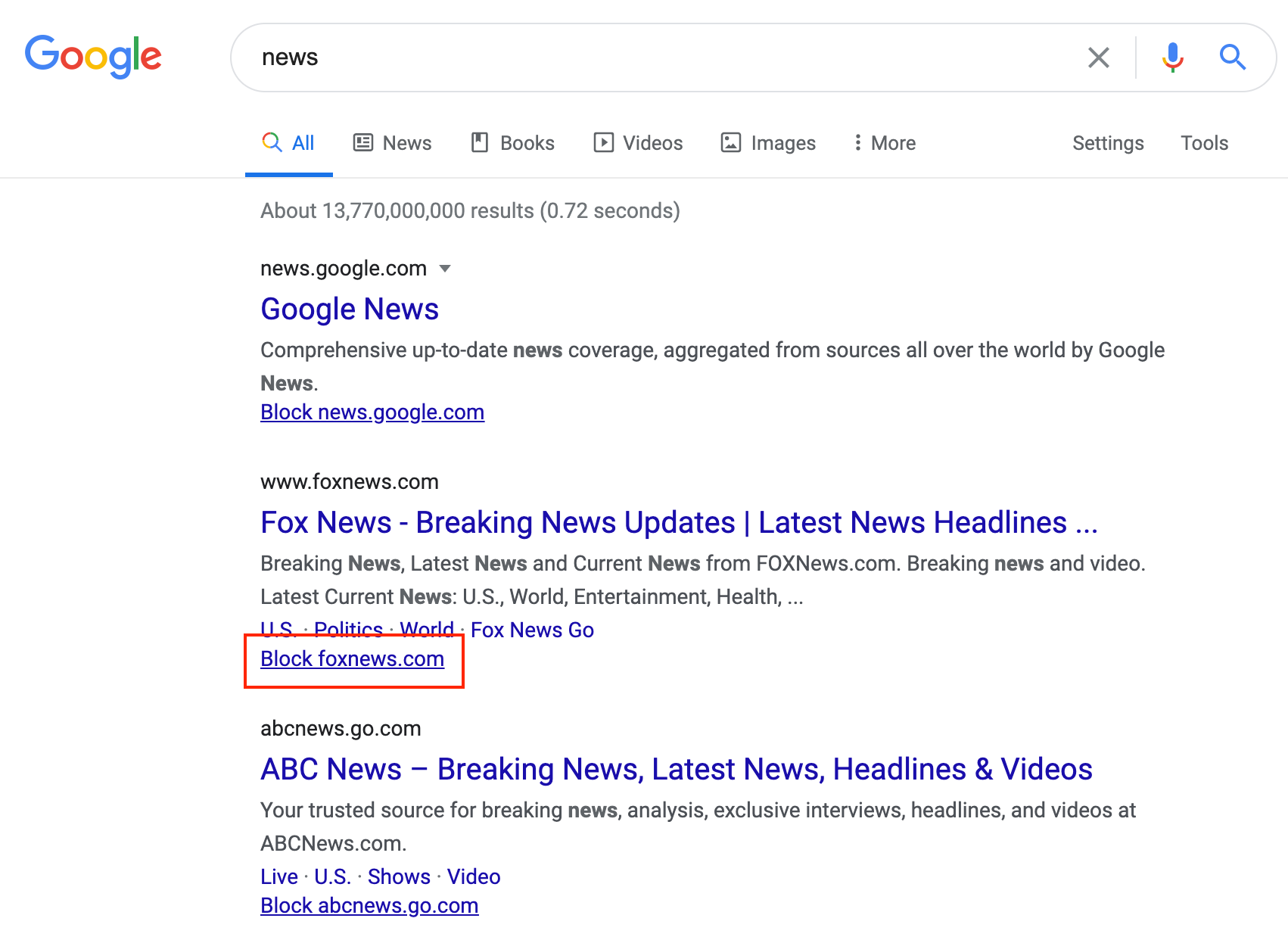The image displays a Google search results page. In the top left corner, the Google logo is prominently placed. Adjacent to it is a long search bar with the word "news" typed in lowercase letters.

Below the search bar, there is a navigation menu starting with the word "All," which is underlined in blue. This is followed by more options: "News," "Books," "Videos," "Images," and "More." Additional settings and tools options are located to the right.

As the search results begin, the first clickable option is "Google News," in blue text with the URL "blocknews.google.com" underlined below it. The next result features "Fox News," highlighted in blue, followed by the description "Fox News, Breaking News Updates, Latest News Headlines." Enclosed within a red outlined box is the text "blockfoxnews.com," also underlined and in blue.

Further down, "ABC News" is listed with a description that reads: "ABC News - Breaking News, Latest News, Headlines, and Videos. Your trusted source for breaking news, analysis, exclusive interviews, headlines, and videos at abcnews.com." The URL "blockabcnews.go.com" is underlined at the very bottom.